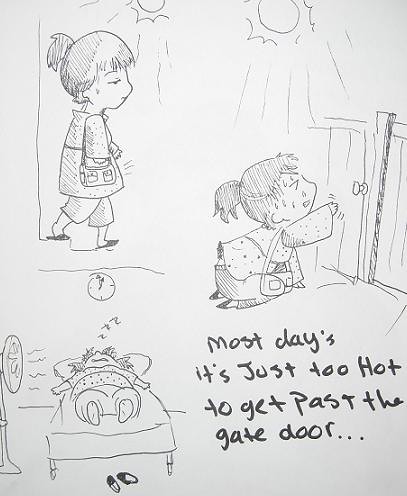The image is a hand-drawn comic strip in shades of black, white, and gray, depicting a young girl struggling with the heat. The top left panel shows the girl walking down the steps of her house, visibly sweating with droplets falling down her face. She wears a jacket, shorts, and a ponytail. The top right panel illustrates her on her knees, reaching for a door knob, looking exhausted under the intense sun that is clearly shown in the image. The bottom left panel portrays the girl laying in her bed, with her shoes on the floor beside her and a fan blowing on her as she sleeps, seeking relief from the oppressive heat. The text at the bottom right states, "Most days it's just too hot to get past the gate door..."